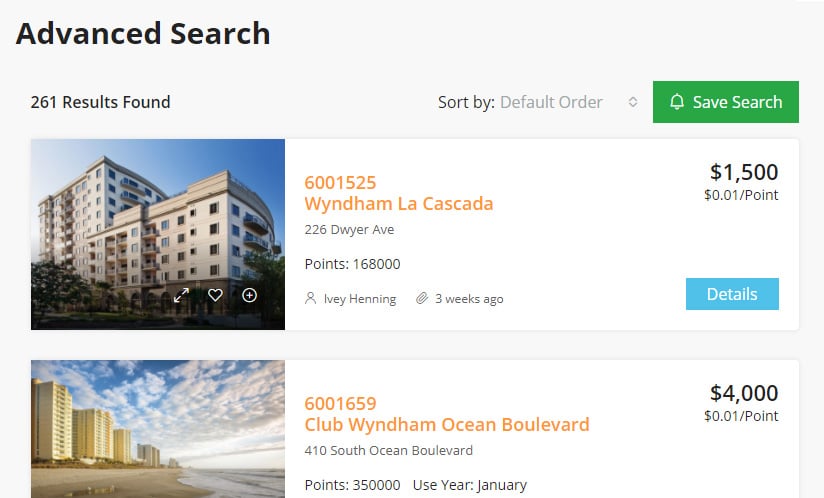The screenshot depicts an advanced search results page displaying a total of 261 results. The page offers sorting options via various filters and includes the ability to save the search using a green button adorned with a bell icon. Two specific listings are visible in this detailed view. The first listing is for "Windham La Cascada," featuring an image of an extensive apartment complex resembling a multi-building hotel, with a price tag of $1,500. A blue "Details" button is positioned at the bottom right of this listing. Below, the second listing is for "Club Windham Ocean Boulevard," located at 410 South Ocean Boulevard, with a luxury price of $4,000. This listing showcases multiple high-rise buildings situated directly along the ocean shore, highlighting a stunning and luxurious beachfront setting.